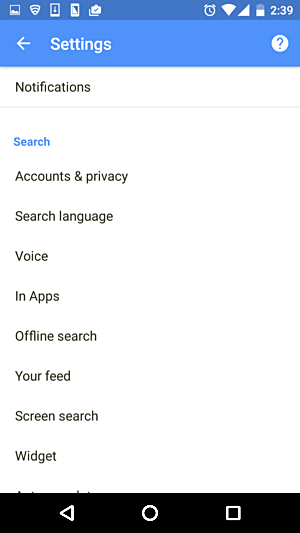A screenshot captures the settings page of an outdated smartphone interface at precisely 2:39 p.m., with the battery indicator showing around 50% remaining. The visual style features a blue, black, and white color scheme, presenting a somewhat antiquated user interface design. Prominent menu options such as "Privacy," "Voice," "Apps," "Feed," and "Widgets" are distinctly visible, hinting at various customization and configuration features available to the user. At the bottom of the screen, a black navigation bar displays three traditional icons: an arrow, a circle, and a square, typically representing back, home, and recent apps functions. The overall aesthetic and functionality suggest it's a straightforward settings menu, devoid of any groundbreaking elements.